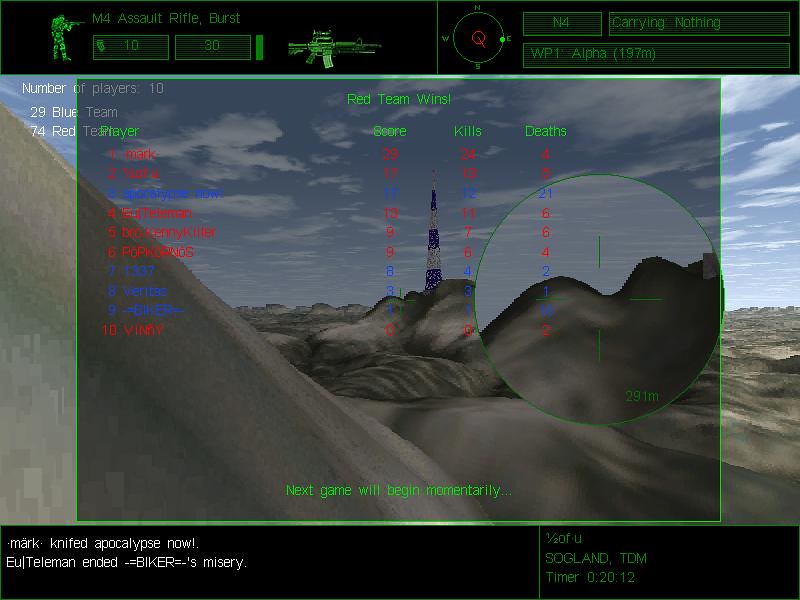In this image from a computer game, the terrain is depicted in various shades of gray, giving it a puffy, cloud-like appearance. Dominating the center of the scene is a striking tower adorned in white and blue hues. The sky above is heavily overcast, contributing to the overall cloudy atmosphere.

The interface indicates that there are 10 players participating. The scoreboard shows the blue team with 29 points and the red team leading with 74 points. At the top of the screen, a bold announcement declares, "Red Team Wins!" in an exclamatory style.

Statistical information is presented in black text across the top and bottom of the interface. Featured prominently on the screen is an image of a player wielding a machine gun, accompanied by a detailed depiction of the weapon itself. A compass is also visible, presumably for navigation purposes.

Additional data indicates that the player is currently carrying no items. A label marked "WP-1 Alpha" is present, possibly indicating a specific location or mission designation within the game. 

The left side of the image reveals a mountainous landscape. A box within the frame lists the stats for each player on both the red and blue teams. Furthermore, a circular panel provides an up-close view of the gray, puffy terrain where the gameplay is unfolding.